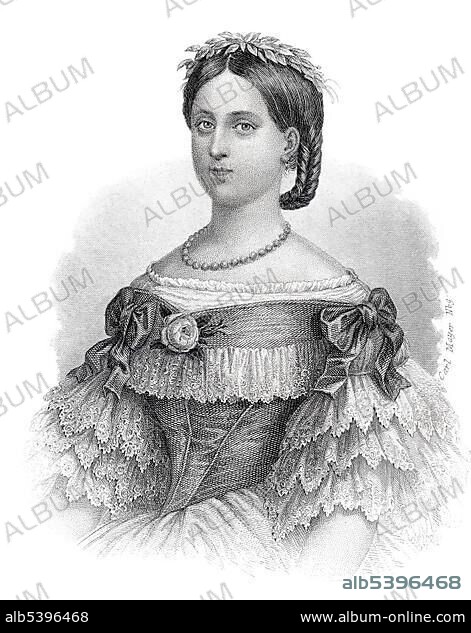This is a black and white drawing of a regal woman dressed in Victorian-era attire. The drawing, sourced from an online album (www.album-online.com), bears the identification number ALB 539-964-68, along with watermarks saying "album" across the entire image. The woman is depicted in a sophisticated old-style dress adorned with ruffles on the sleeves and across the bustline. She wears a pearl necklace and her hair is parted in the middle, intricately braided, and looped around the back. On her head, she dons a laurel headpiece crafted from leaves. Her neckline, adorned with a rosette, is elegant yet conservative. The woman is looking sternly straight ahead, adding a sense of seriousness to the portrait.